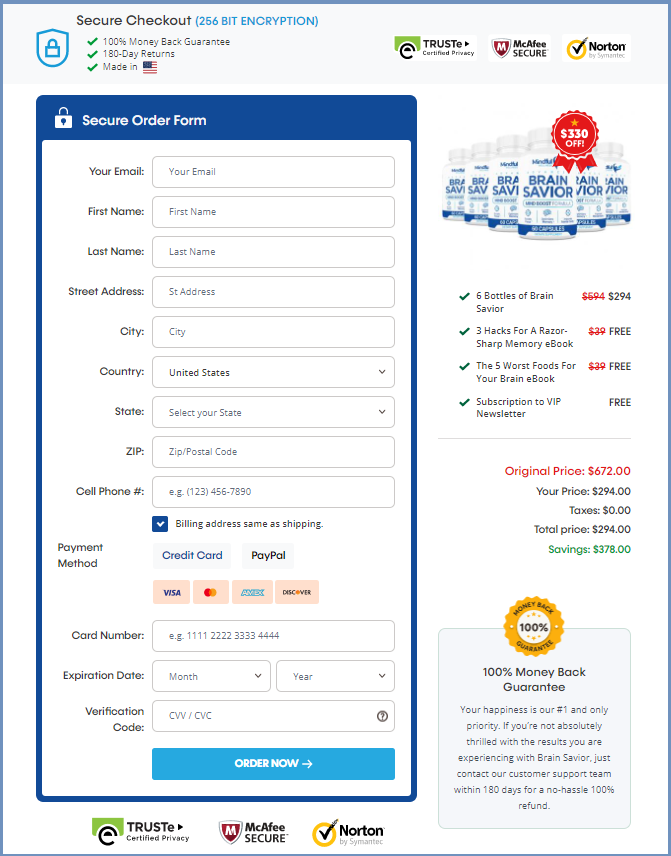This screenshot captures the secure checkout page of a website, designed to reassure customers of its safety features. The background uses an off-white color, contributing to a clean and inviting look.

At the very top left corner, the phrase "Secure Checkout" is prominently displayed in black font. Adjacent to it, in blue font, is the reassurance text "(256-bit encryption)." Directly below this section, there is a blue shield icon featuring a lock symbol, signifying security.

To its right are three red vertical checkmarks, each paired with a trust-building statement: 
1. "100% Money-Back Guarantee"
2. "180-Day Returns"
3. Accompanied by an American flag icon, the phrase "Made in USA"

On the right side of this area, three security logos are presented: 
- TrustE
- McAfee Secure
- Norton Antivirus, marked with a checkmark

Beneath this, a blue-outlined vertical rectangle highlights the text "Secure Order Form" in white font at the top. The form includes numerous fields for inputting personal information: email, first name, last name, street address, city, country, state, zip code, cell phone number, and an option checkbox for "Billing address same as shipping." 

This detailed layout effectively communicates the website’s commitment to security and customer satisfaction.